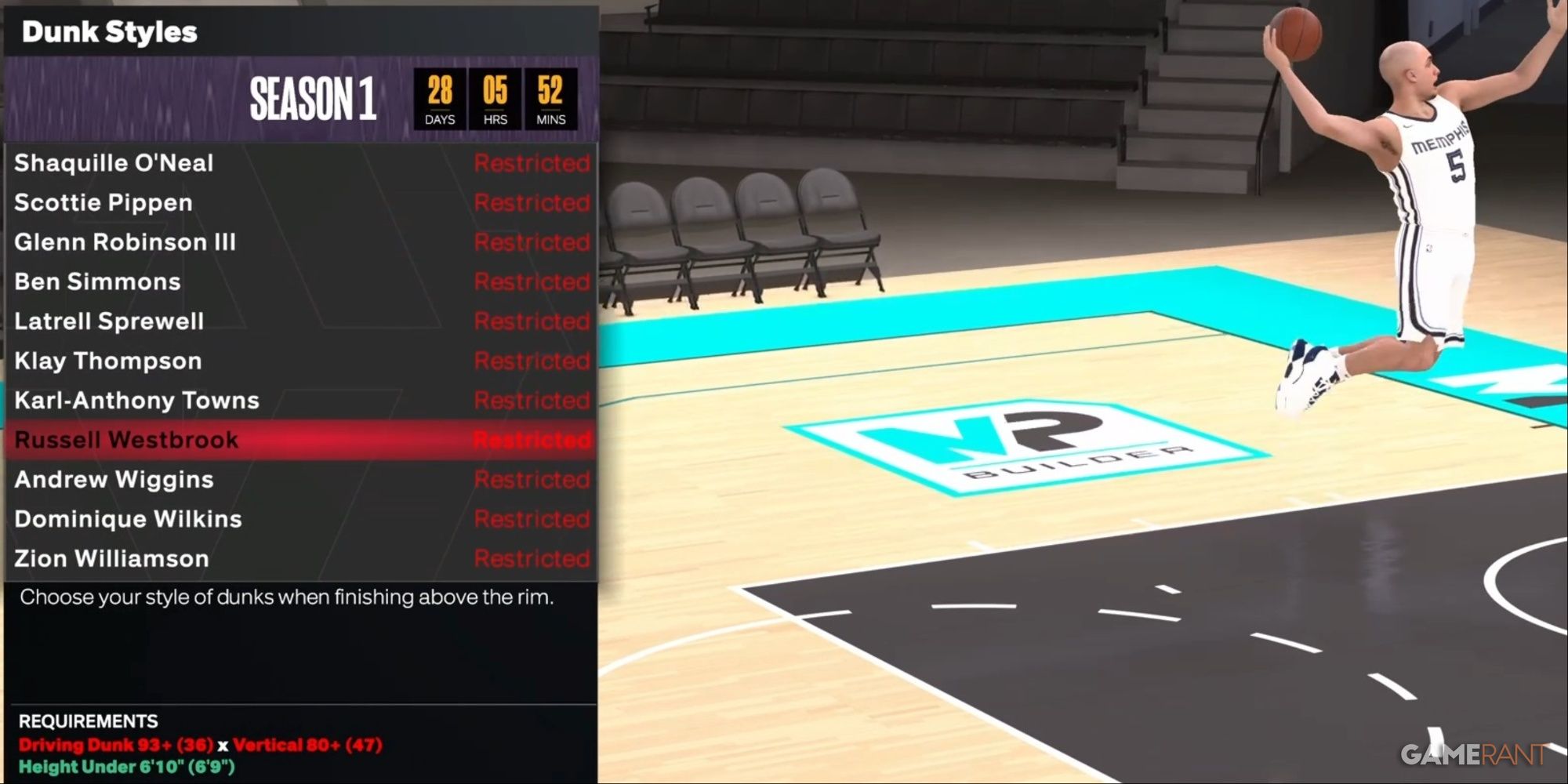The image appears to be a screenshot from a basketball-themed video game titled "Dunk Styles: Season 1." The focus of the image is a basketball player from the Memphis team wearing a white uniform with the number 5 on his jersey. The player is captured mid-air, holding a basketball in his right hand, poised for a slam dunk. Although the basketball hoop isn't visible, the player's dynamic pose suggests he is about to execute a powerful dunk.

To the right, there's a depiction of a half basketball court featuring the logo "MP Builder," which for this context, might indicate a sponsor or specific game mode. The court is detailed with elements typical to a basketball arena, including chairs along the sideline and stairs leading up to spectator seating. The floor features a sophisticated design with shades of blue and black, underscored by high-quality graphics that clearly identify this as a realistic video game render rather than a photograph.

On the left side of the image, there's a detailed roster list under the "Dunk Styles: Season 1" banner, highlighting famous NBA players such as Shaquille O'Neal, Scottie Pippen, Glenn Robinson III, Ben Simmons, and many others, with Russell Westbrook's name highlighted and marked as "Restricted." The section also includes requirement statistics for players, indicating necessary height and attributes with figures displayed in red and green. The gameplay details seem to emphasize choosing specific dunk styles and meeting certain criteria to unlock or play with various players.